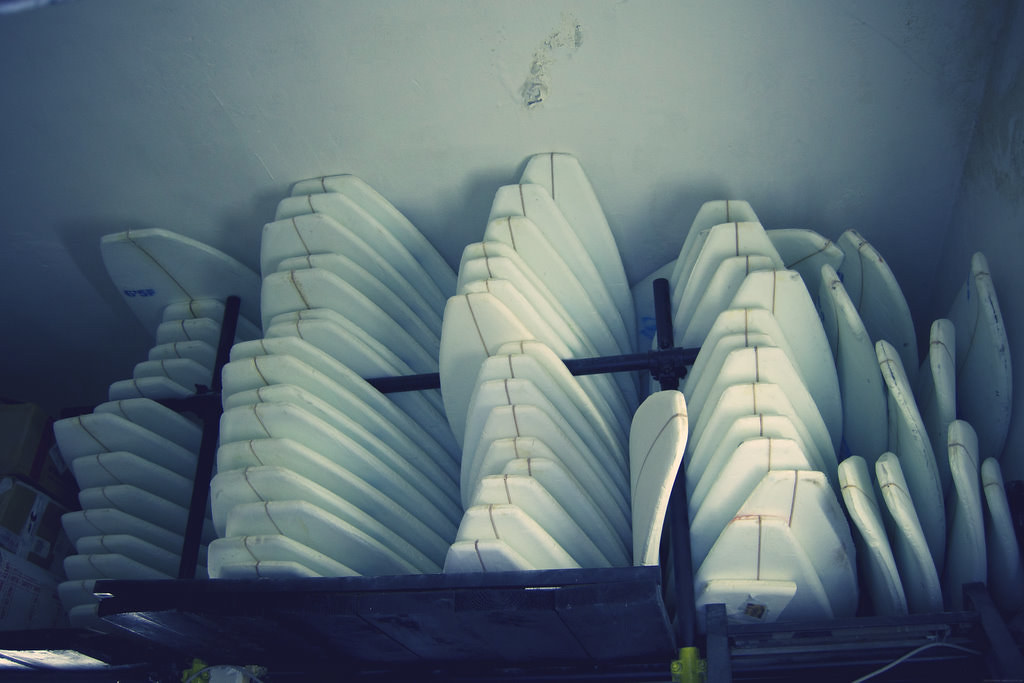The image shows a dimly lit scene featuring a series of white, curved boards that are likely some form of recreational or sport equipment, possibly surfboards, skateboard blanks, or water skis. These boards are arranged vertically from top to bottom within a metal frame holder or rack. In front of the rack is a large metal fence, connected by numerous metal bars ending with yellow caps. The boards have a slight upward curve and vary in shape, some being pointier while others are broader. The far wall in the background is white and has a noticeable chip in the center, with some of the paint peeling off. The overall scene lacks vibrant colors, emphasizing the stark contrast between the white boards and their metal surroundings.